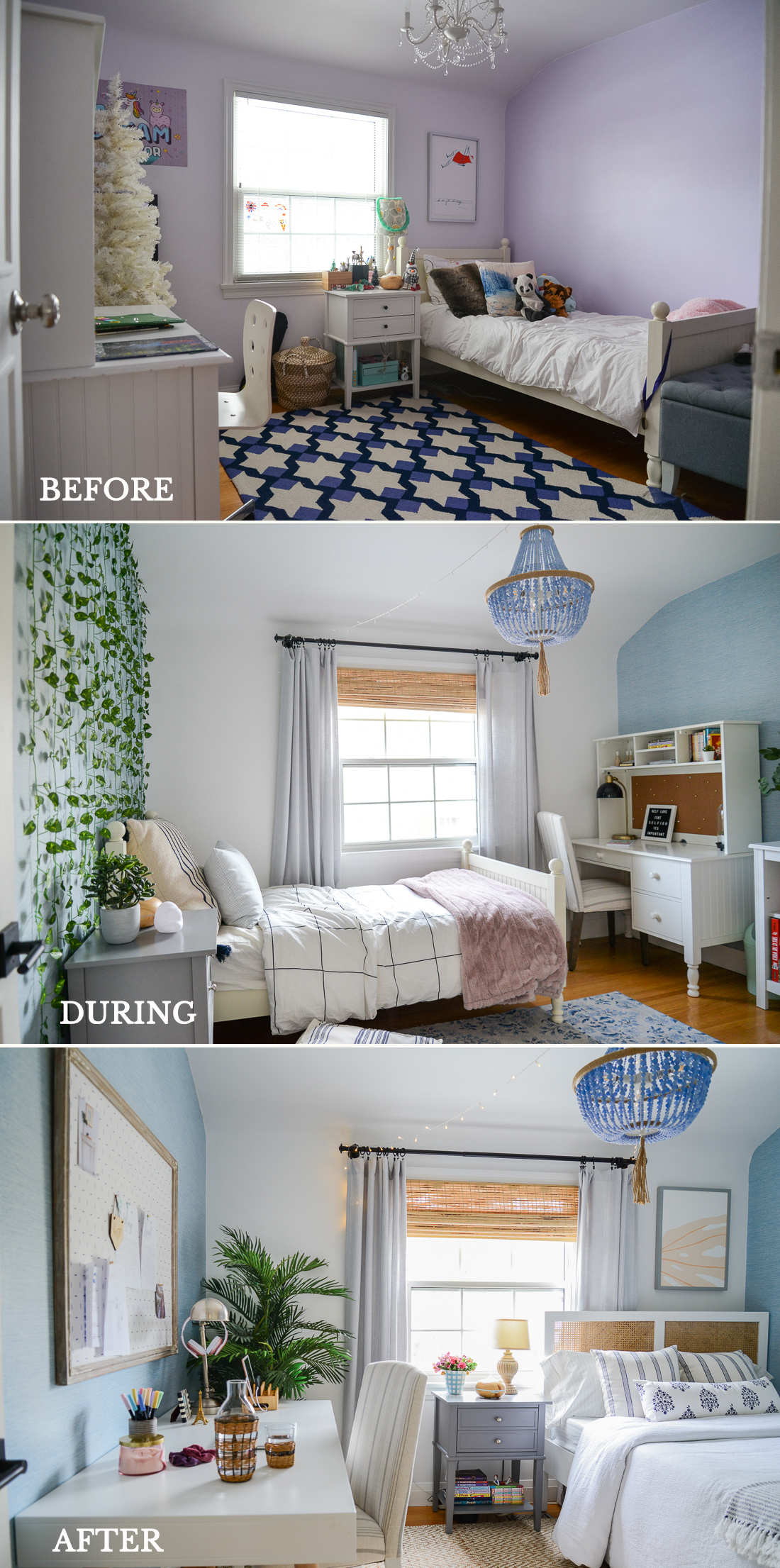This set of three images captures the transformation of a bedroom from its initial state through a renovation process to the final look. The "before" picture at the top features a room with pinkish-purple walls, a small wooden bed with a white mattress and blanket positioned against the right wall. A blue, white, and black star-patterned rug is spread on the floor. An elegant chandelier is fixed to the ceiling, and there's a wooden desk with various accessories in the room. The "during" photo in the middle shows significant changes: the walls are now painted white with green vine decals, and the bed is repositioned to the left wall. A white desk with a corkboard inset appears against the wall where the bed used to be, and grey furniture, including a dresser, is introduced. The "after" image at the bottom depicts the final arrangement with the bed moved back to the right side, adorned with a white blanket and blue and white pillows. The room now features added green plants, a white chair, and a redesigned workspace. The window remains constant across all images, with consistent curtain rods and curtains, providing a cohesive element throughout the transformation.